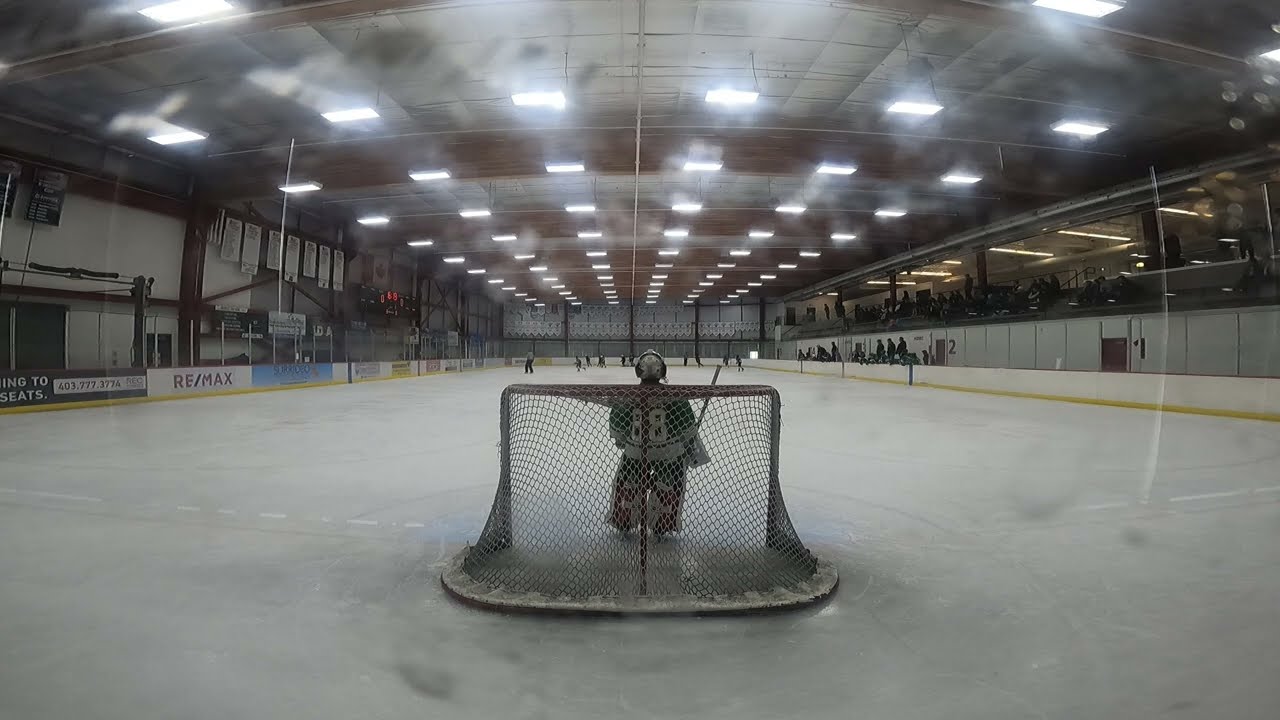This photo captures the scene at an indoor hockey rink from behind a glass partition, focusing on a lone goalie. The young goalie, who appears to be fairly short and possibly a kid, stands in the net wearing the number 88 on a green jersey and a white hockey mask. The arena, likely an amateur or semi-professional setup, is spacious with noticeable warehouse-style ceilings. The ice rink is illuminated by bright lights, which, combined with the glare from the glass, give the image a somewhat hazy appearance. On the left side of the photo, an advertisement for REMAX is visible on the wall. In the far distance, other hockey players and some spectators are barely discernible on the ice and sitting in the stands on the right side, emphasizing the goalie’s isolation in the foreground.